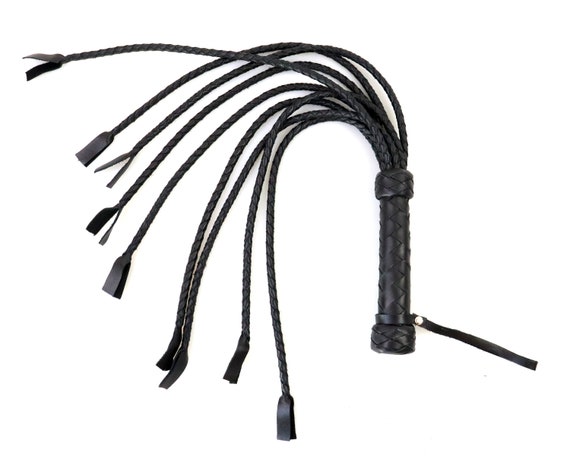In the image, set against a completely white background, there is a prominently featured black leather object, which appears to be a whip or flogger. The object is positioned to the right side of the image. The handle, at the bottom, is sturdy and wrapped with a nylon-cord-like material, giving it a braided appearance. Around this handle is a band with two small knobs, from which a black strap extends downward and to the right. The top of the handle has another band resembling a napkin holder, and from it, several braided cords emerge and fan out to the left. There are eight or nine of these cords, some curving and some extending straight to the left. Each cord appears to have flat rectangular ends, with some possibly splitting into two at their tips. Overall, the meticulously detailed object lies flat, showcasing its structured and elaborate design.